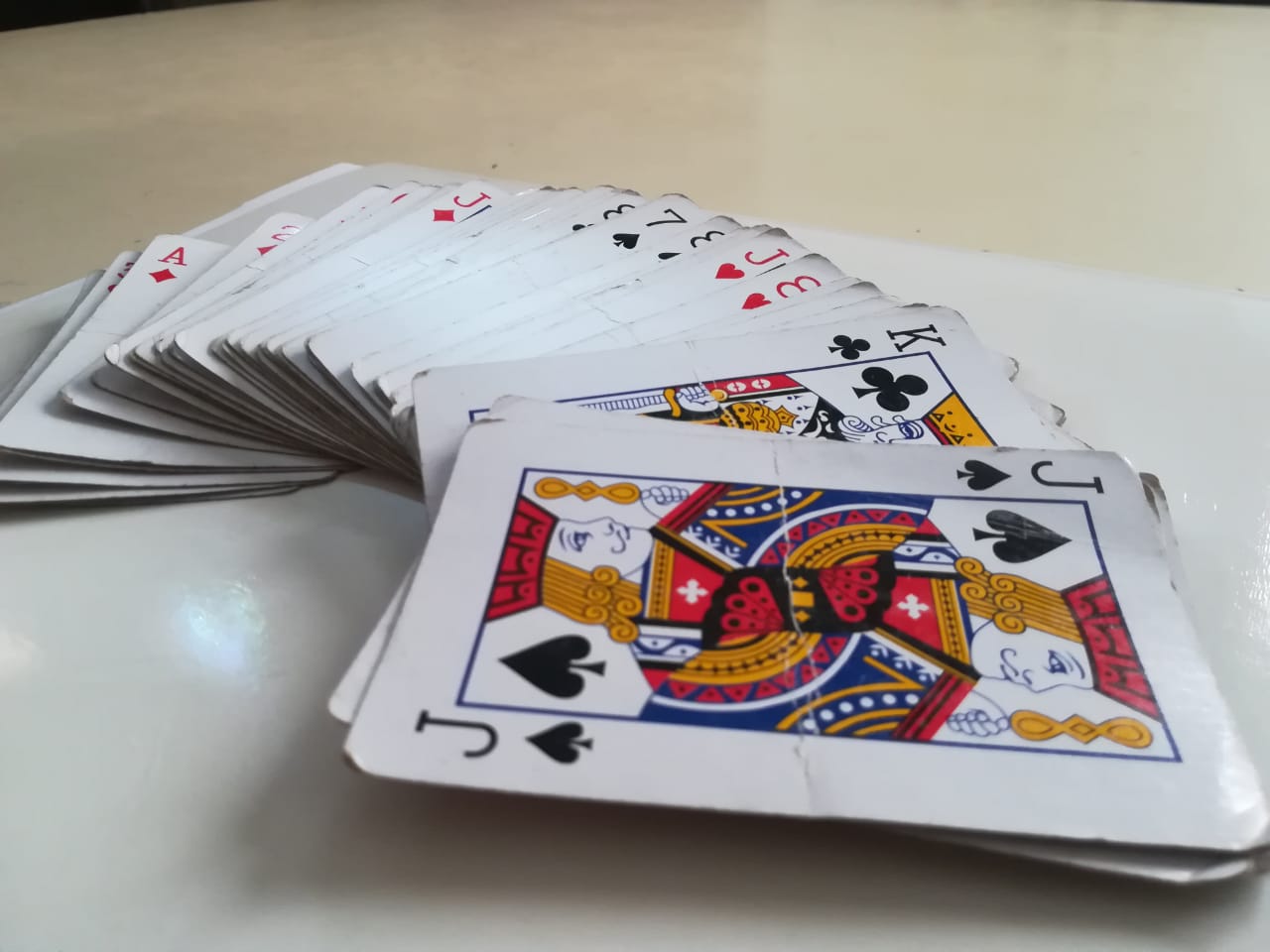A slightly disheveled deck of playing cards is spread out, with most of the cards partially overlapping each other. Prominently visible at the top of the arrangement is the Jack of Spades, displaying a classic, old-fashioned design with vibrant colors highlighting the royalty. The cards rest on a light brown table, which appears to have a poster board beneath it. The deck shows signs of extensive use; many cards are creased, with bent corners and smudges indicating frequent handling. This well-worn look suggests the cards have been used not just for casual play, but also for performing tricks or skillful dealing. Among the visible cards, there is an Ace of Diamonds and a King of Clubs, adding to the spread's eclectic appearance.